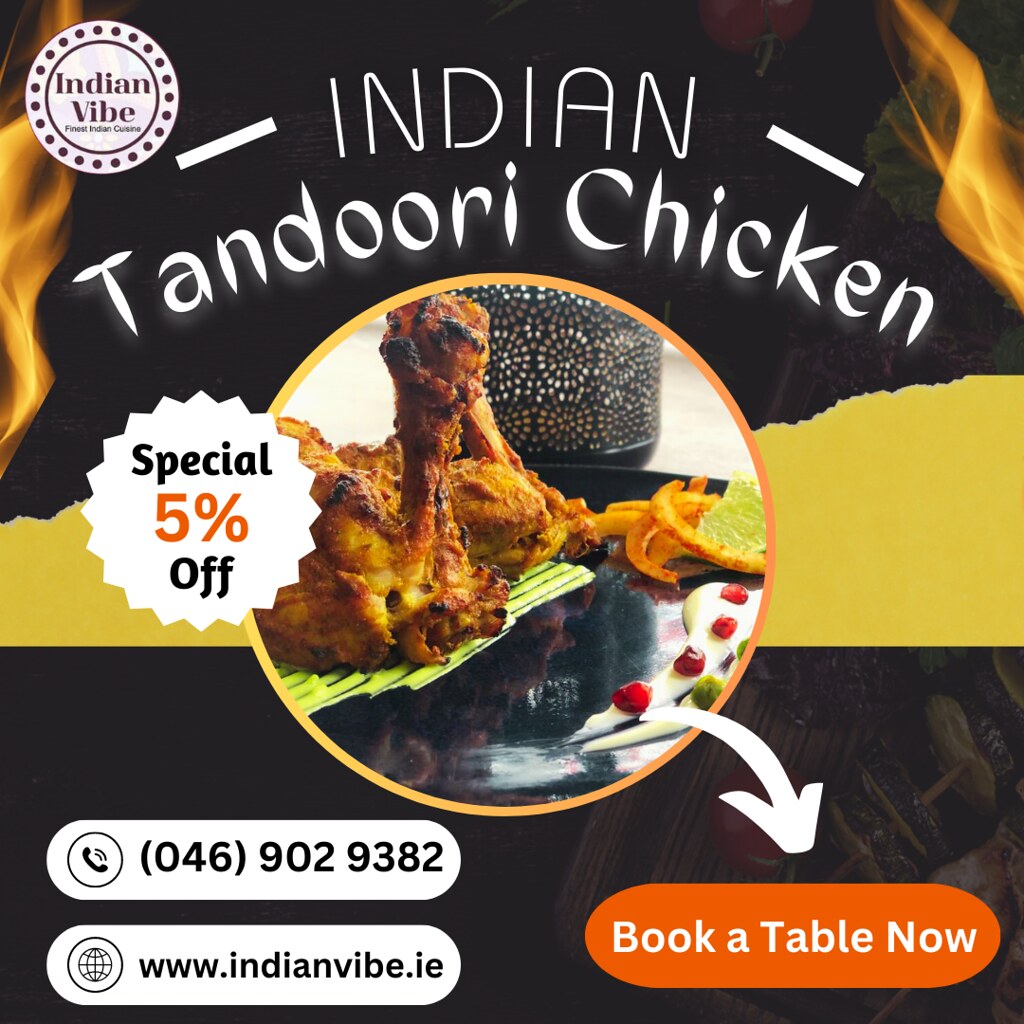This is an online advertisement for the restaurant Indian Vibe, specializing in Indian Tandoori Chicken. The square, Instagram or Facebook-style graphic is visually striking with a central circular image of a plate of tandoori chicken with fried onions and a lime slice. A notable feature is a jagged-edged white badge overlapping the chicken image, announcing a "Special 5% Off." The dark background features flames on the left and right sides, enhancing the spicy appeal of the dish.

At the top left, a circular logo with dots around the edge reads "Indian Vibe, Finest Indian Cuisine." The title "Indian Tandoori Chicken" arches over the central image in bold, white text. Cutting through the middle of the ad is a thick, yellow strip that contrasts sharply with the black sections at the top and bottom.

In the bottom left corner, contact information is conveniently provided in white rectangles: the phone number 046-902-9382 and the website www.indianvibe.ie. On the bottom right, an orange rounded rectangle with white text and an arrow pointing downwards invites viewers to "Book a Table Now."